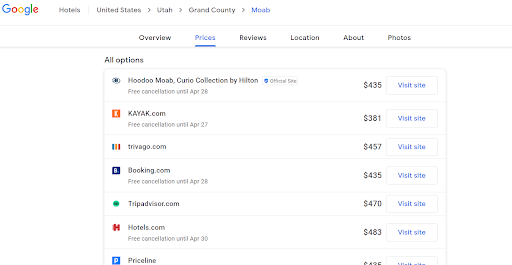The image appears to be a screenshot of a Google Hotels search results page focused on Grand County, Utah, in the United States. The screenshot is small, making the details somewhat difficult to discern. The page lists seven different hotel options, with their respective prices ranging from approximately $380 to $450 per night. Each listing includes clickable links to visit individual hotel websites for further information. The prices suggest that these are mid-range to higher-end accommodations. Overall, this screenshot is a captured summary of available hotel choices in the specified region, intended to aid in travel planning.